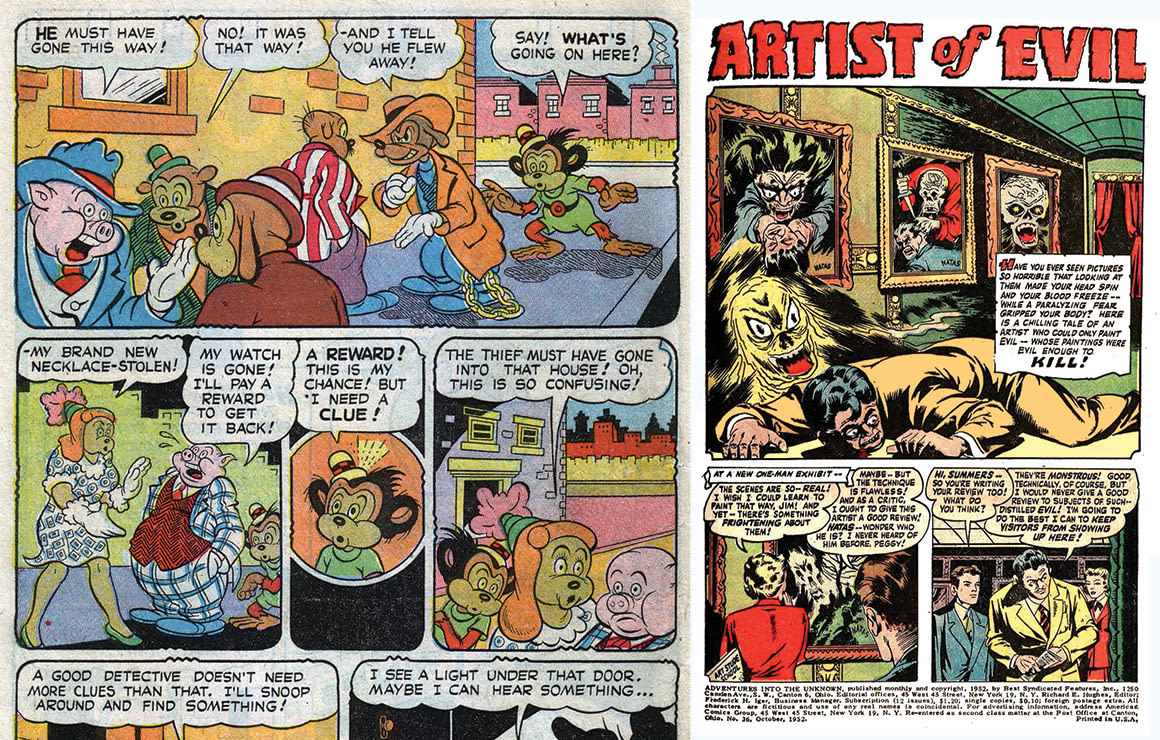This image depicts a page from a vibrant, classic-style comic book. The top left panel features a colorful ensemble of animal characters dressed as gangsters, including a pig in a blue suit and hat, a green-jacketed bear, a walrus in a red and white striped jacket, and a monkey. They are in the midst of a conversation, with the pig pointing and saying, "He must have gone this way," while the bear retorts, "No, it was that way." A dog chimes in, "And I tell you, he flew away," as the monkey interjects, "Hey, what's going on here?"

The next panel below shows a commotion involving theft victims. A female character in a white and blue dress exclaims, "My brand-new necklace, stolen!" A pig in a checkered blue and white suit adds, "My watch is gone. I'll pay a reward to get it back." The nearby monkey overhears and thinks, "A reward. This is my chance, but I need a clue."

Continuing their eavesdropping, the monkey picks up more clues from the conversation. Another character suggests, "The thief must have gone into that house. Oh, this is so confusing." The determined monkey muses, "A good detective doesn't need more clues than that. I'll snoop around and find something. I see a light under that door. Maybe I can hear something."

On the right side of the page is a separate strip titled "Artist of Evil," depicting dark, ominous scenes with monstrous creatures and worried characters, contributing an eerie contrast to the vibrant gangster mystery playing out on the left.